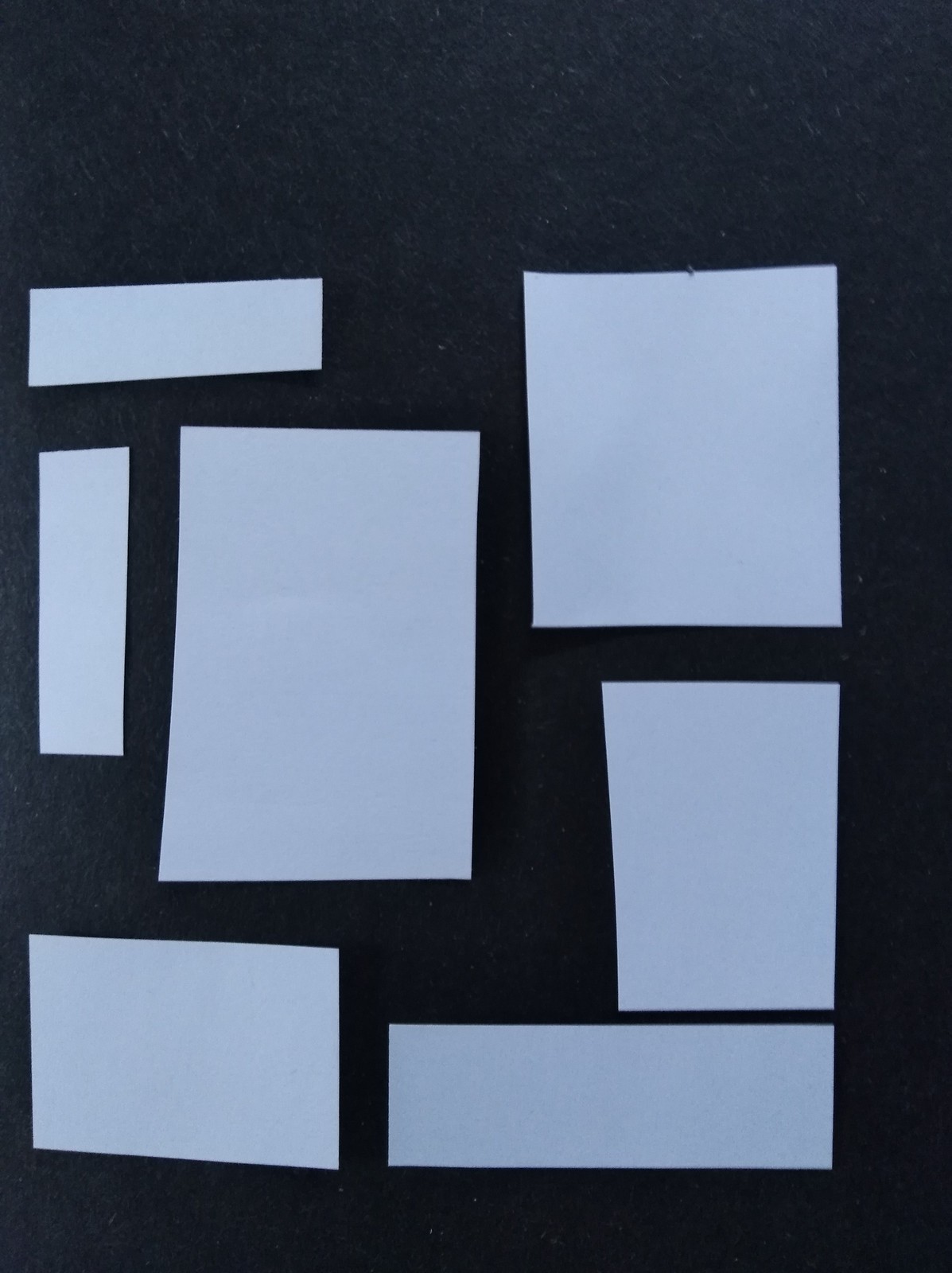A meticulously crafted abstract composition, likely computer-generated, showcases a series of rectangles against a predominantly black background with subtle hints of white static. In the top left corner, a small, horizontal pale blue rectangle is positioned above a slightly larger vertical rectangle, although the two do not touch. Moving to the right, a significantly larger vertical rectangle stands prominently. Below it, an almost square-shaped figure rests horizontally. In the upper right quadrant, another near-square sits vertically aligned. Directly beneath it is yet another vertical rectangle, and beneath this, a long horizontal rectangle stretches across the frame. Altogether, the seven distinct pale blue rectangular and near-square shapes float independently within the composition, creating a balanced yet dynamic visual arrangement.